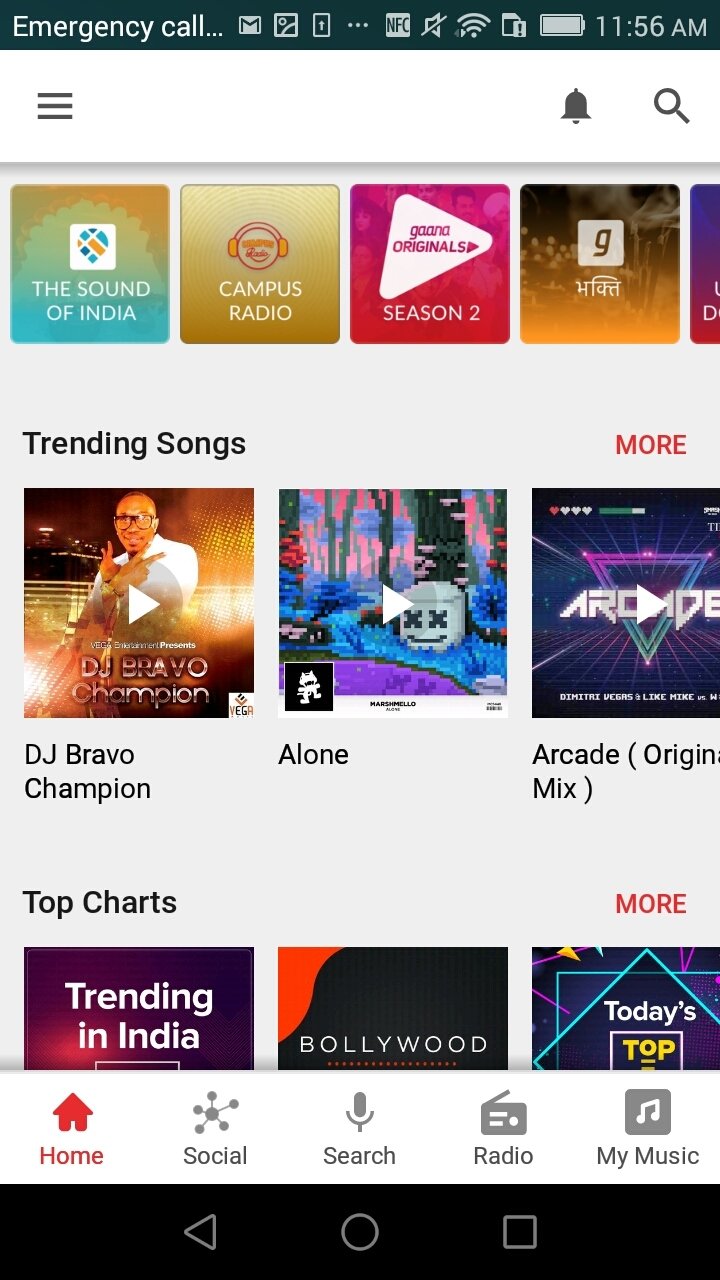In this image taken from a cell phone screen, the top section features a black rectangle with "Emergency Call..." prominently displayed. This area also contains several symbols including a photo icon, miscellaneous other icons, and a trio of horizontal dots. The speaker is shown as muted, the battery icon appears fully charged, and the time is clearly indicated as 11:56 a.m. 

Beneath this top bar, there is another section with black horizontal lines, a bell icon on the right for notifications, and a magnifying glass icon for search. The main content area starts with clickable icons labeled "The Sound of India," "Campus Radio," "Something Season 2," and a partially visible "G."

Further down, a section marked "Trending Songs" lists tracks such as "DJ Bravo Champion," "Alone," and "Arcade Original Mix." Continuing to scroll reveals a "Top Charts" area featuring categories like "Trending in India" and "Bollywood." 

At the bottom of the screen, a navigation bar includes several icons: Home, Social, Search, Radio, and My Music.